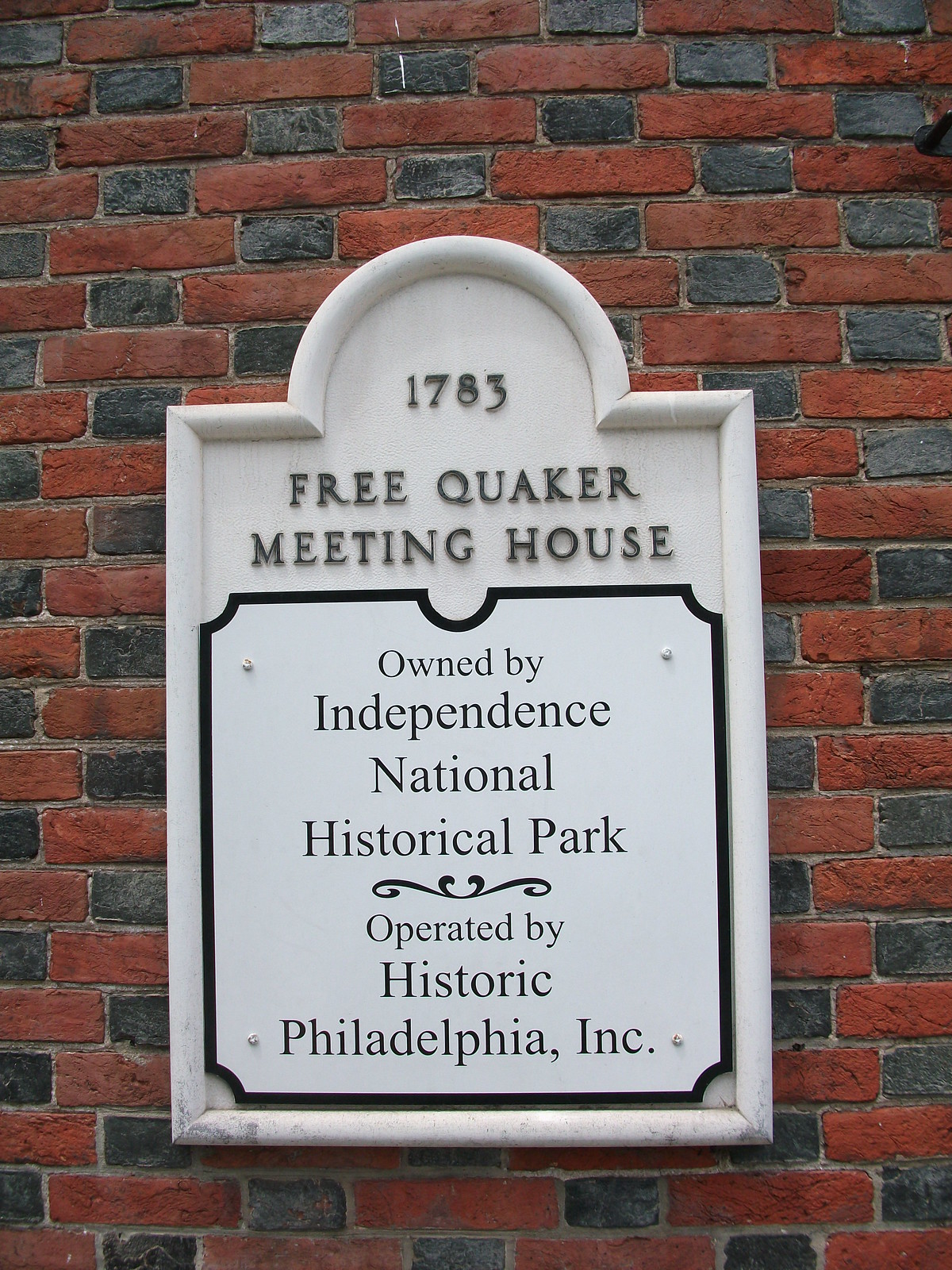The image is a color photograph in portrait orientation, depicting a rust-colored and grayish-green brick wall forming an organized pattern. At the center of the image is an ornate historical sign, characterized by a white background and black text. The layout of the sign is rectangular with a semi-circle at the top. The semi-circle contains the date "1783," followed by the inscription "Free Quaker Meeting House" beneath it. Underneath this, the sign states that the property is "Owned by Independence National Historical Park" and "Operated by Historic Philadelphia, Inc." A swirly logo separates these lines of text. The sign's ornate design is complemented by a black border around the center part.